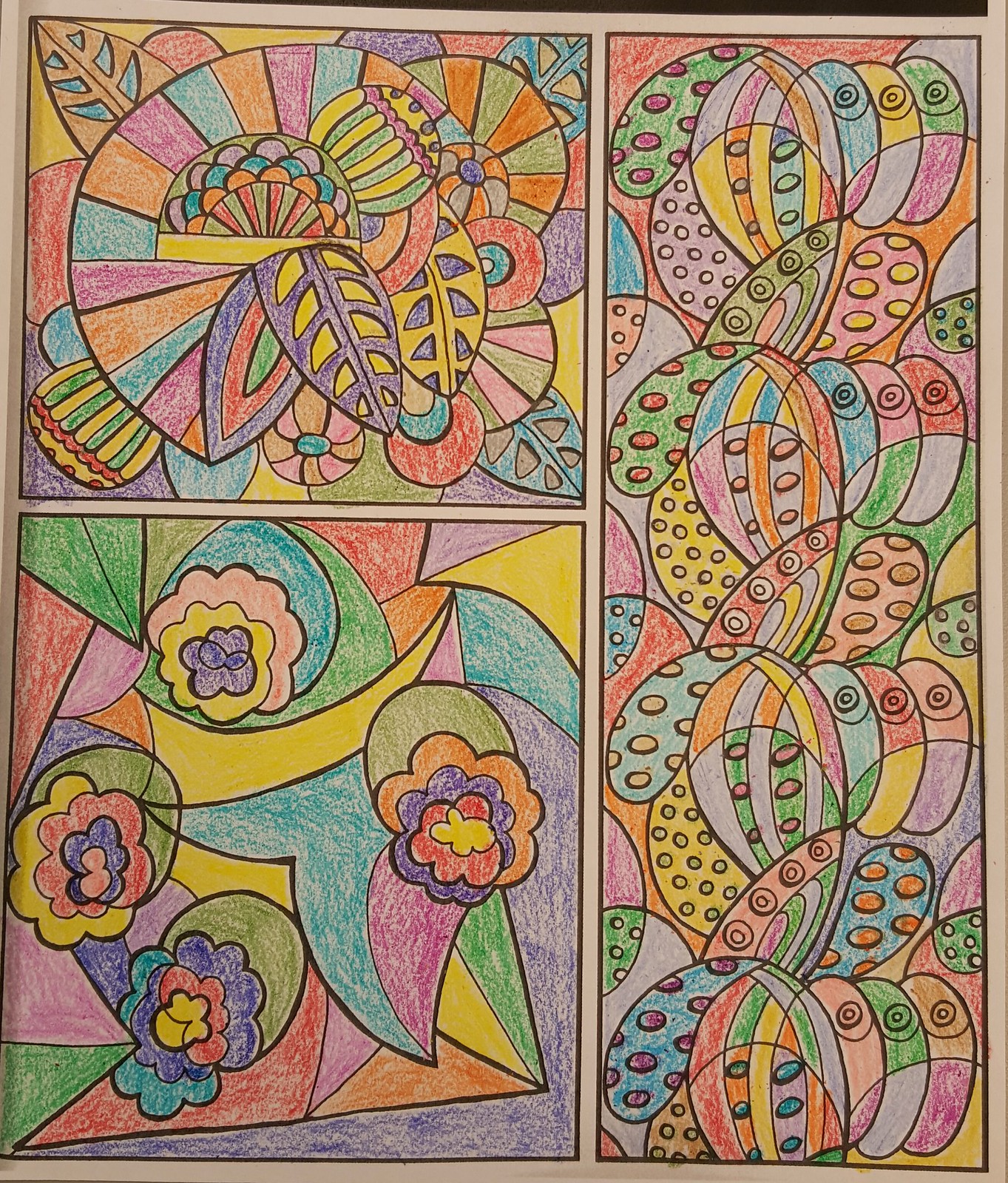This image portrays a vibrantly colored page that appears to be from an adult coloring book, meticulously filled in with either crayons or colored pencils. The page features a variety of abstract shapes, including the top of a hot air balloon, half-circles, cut-off triangles, and what resembles the top of a jester's hat. It also includes swirling shapes that evoke the appearance of cacti adorned with circles of varying sizes. The color palette is rich and extensive, incorporating purples, blues, oranges, yellows, greens, reds, and pinks. 

The page is completely colored in, with every section neatly filled, suggesting the work of an adult or someone with notable artistic skill. The finished page, possibly torn out or still within the book, shows a faint off-white border that frames the intricate designs. The combination of floral elements, leaves, and patterned shapes creates a cohesive and visually engaging composition.